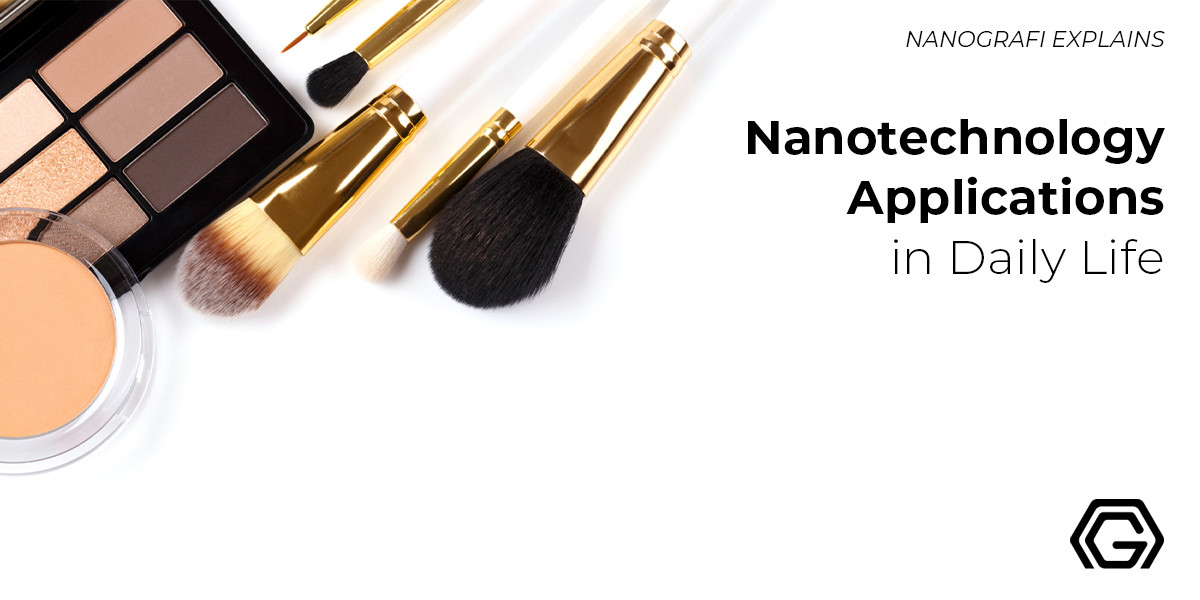The image features a pristine white background. Dominating the upper right corner, in bold black font, is the title "Nanography Explains." Below this, also in bold, reads "Nanotechnology Applications," followed by the lighter text "In Daily Life." On the bottom right, there is a distinct logo—a hexagram with a 'G' nestled inside it, although the bottom part of the hexagram is cut off from view.

To the left-hand side, a variety of makeup items are displayed. In the upper left, there is a palette of eyeshadows in various shades of tan and brown, oriented at a 45-degree angle counterclockwise. Below it, a partially visible compact in fleshy peach tones peeks out, accompanied by five makeup brushes of varying sizes. These brushes are arranged diagonally with their bristles pointing downward toward the center of the image, growing in size as they move outward, except for one that is intermediate in length.